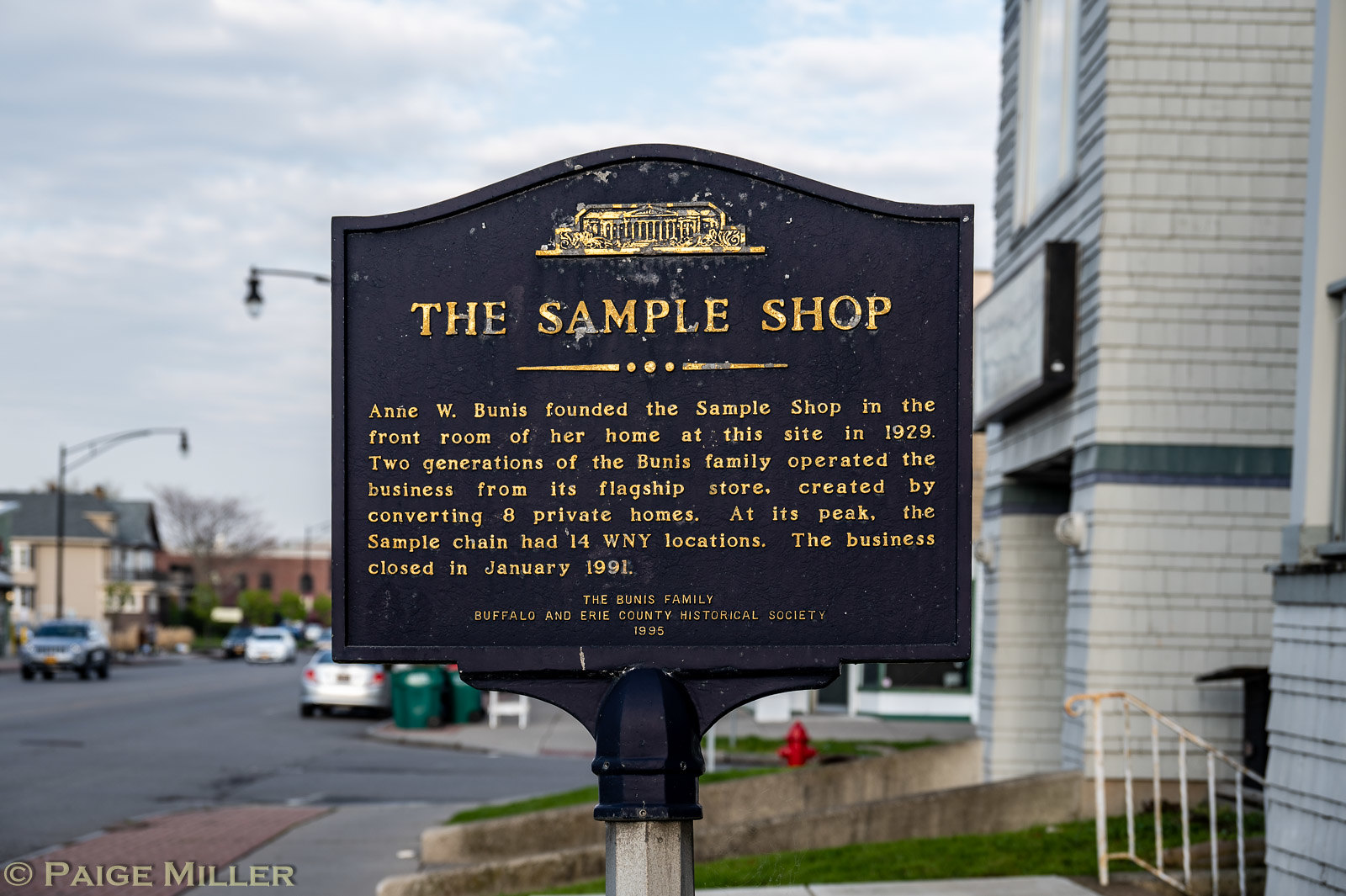This photograph captures a close-up view of a black metallic sign, mounted on a pole, in an urban outdoor setting. The sign bears gold lettering with the title "The Sample Shop" prominently displayed at the top. Below the title, there is a detailed paragraph narrating the history of the shop: "Anne W. Bunness founded The Sample Shop in the front room of her home at this site in 1929. Two generations of the Bunness family operated the business from its flagship store created by converting eight private homes. At its peak, the Sample chain had 14 WNY locations. The business closed in January 1991." The close-up nature of the photograph means the entire pole isn't visible.

In the background, a bustling cityscape is evident. On the left side, a road is busy with moving cars, parked vehicles, and a house across the street. Streetlights line the sidewalk, which ends with visible garbage cans. Further left, some brick buildings can be seen in the distance. To the right, there is a prominent gray structure, potentially a parking garage, complete with a cement ramp. Above, the sky is a patchwork of blue and clouds. At the bottom left corner of the image, a watermark reads, "Copyright Paige Miller."